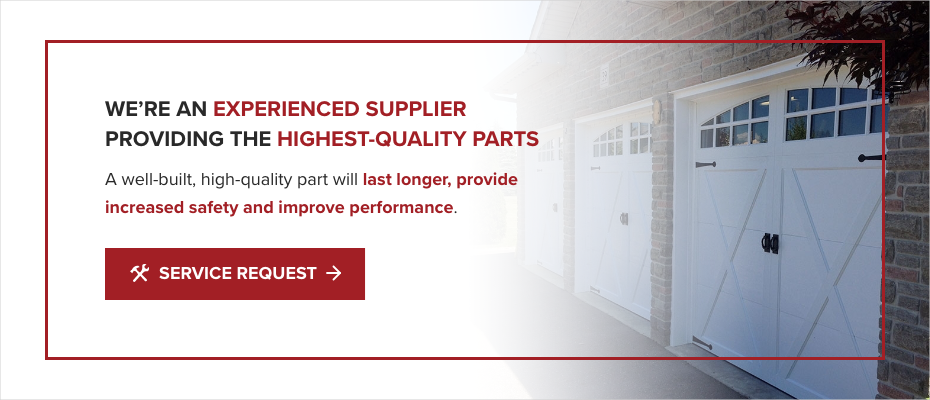The image, sourced from a webpage advertisement, is divided into two distinct sections. On the left, the background is plain white, allowing the text to stand out. On the right side, there is a clear depiction of the side of a house, showcasing three closed garage doors. Each door features windows at the top and decorative X patterns on the lower sections, resembling farm doors, all painted white.

Framing the main content of the advertisement is a red rectangle, inset by about an inch or two, providing a bold boundary. Within this rectangle, black and red text announces, "We're an experienced supplier providing the highest quality parts. A well-built high-quality part will last longer, provide increased safety, and improve performance." Key phrases such as "experienced supplier," "highest quality parts," and "last longer, provide increased safety and improve performance" are highlighted in red for emphasis.

Additionally, there's a prominent red box labeled "Service Request," with white text inside. Adjacent to this, an arrow points to the right, leading towards a graphical representation of tools, signifying a tutorial or further action. This well-organized layout uses color contrast effectively to draw attention to critical information and calls to action.